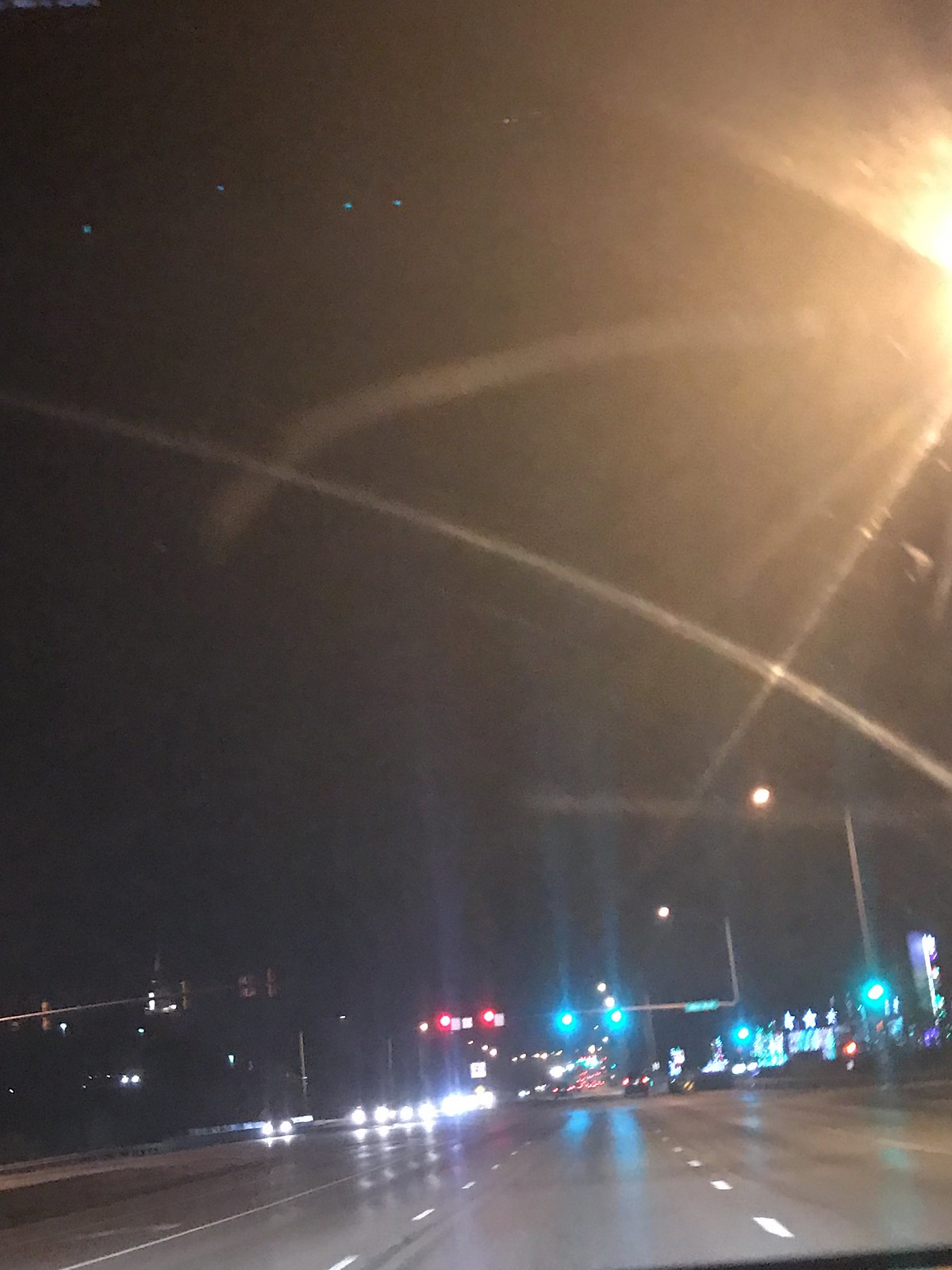This image captures a nighttime street scene taken from inside a vehicle. The perspective is down the center of a wide, multi-lane road, showing a windshield with visible glare and streaks, likely from a windshield wiper. The sky above is pitch black, punctuated by four to six small, blurry blue lights in the top left corner, whose exact nature is unclear due to the low resolution of the image. 

Street lights are visible, with those to the left emitting red light and those to the right a blue-white hue. An intersection is up ahead, with the green traffic lights appearing blue due to image quality. To the top right, a bright orange overhead street light creates significant glare. 

There are several cars on the road, both near and in the distance, with headlights visible from oncoming traffic. The road itself includes a left turn lane and three lanes going straight, with the vehicle positioned in the center of the three straight lanes, around 50 feet from the intersection. Farther ahead and to the sides, dimly lit structures like a gas station and other low-lying businesses can be seen, adding context to the urban setting. The plane of the road appears slightly tilted, enhancing the dynamic feel of this nighttime urban scene.